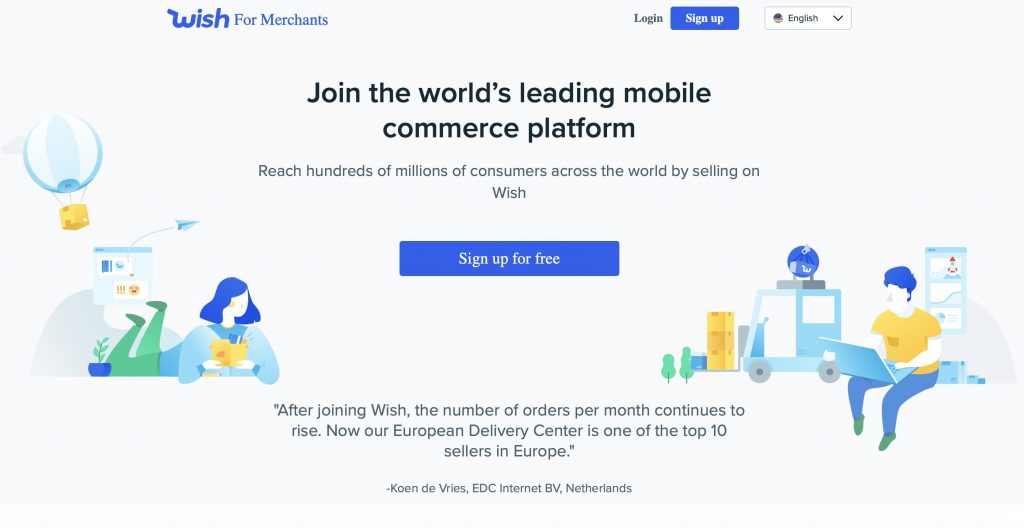The image showcases a promotional page for "Wish for Merchants." Dominating the page is a headline stating, "Join the world's leading mobile commerce platform," accompanied by a descriptive text urging merchants to "Reach hundreds of millions of consumers across the world by selling on Wish." 

The interface features a "Login" button and a "Sign Up" button, the latter highlighted against a blue background. A prominent purple "Sign Up for Free" button offers an inviting call to action. Below this button, gray text provides a testimonial: "After joining Wish, the number of orders per month continues to rise. Now, our European delivery center is one of the top 10 sellers in Europe." The testimonial is credited to "Condevers, EDC, Internet BB, Netherlands," written at the bottom of the page.

The visual design includes a variety of whimsical sketches. One illustration depicts a hot air balloon with a blue circle and a yellow square attached to it. Another sketch features a web page with an arrow, stylized to resemble a blue paper plane. Additional drawings include a person lying on their stomach, apparently holding a yellow dog, with blue hair, and another of a person seated with a laptop on their lap, dressed in a yellow shirt, blue pants, green shoes, and also sporting blue hair.

All these elements are set against a clean white background with black text, creating a visually engaging and informative page.